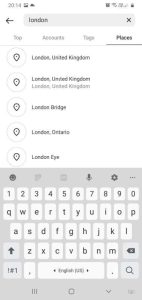This is a low-resolution screenshot taken from a mobile device, likely an iPhone. The image is grainy, making most of the text on the screen difficult to read. At the top of the screen, there's a navigation bar that features an arrow pointing left, suggesting a back button, next to a light gray search bar. The search bar appears to have the word "london" typed in lowercase letters, though the blurriness makes it hard to be certain. To the left of the search bar, there is an X button, which allows the user to clear the search input.

Below the search bar is a navigation menu with several categories. The first category on the left likely says "Top," followed by "Accounts," then possibly "Tags," and finally "Places." In the main body of the screen, under the "Places" category, several location suggestions are listed, each preceded by a map pin icon. The suggestions include "London, United Kingdom," another entry for "London, UK," "London Bridge," "London, Ontario," and "London Eye." At the bottom of the screen is the on-screen keyboard of the mobile device.